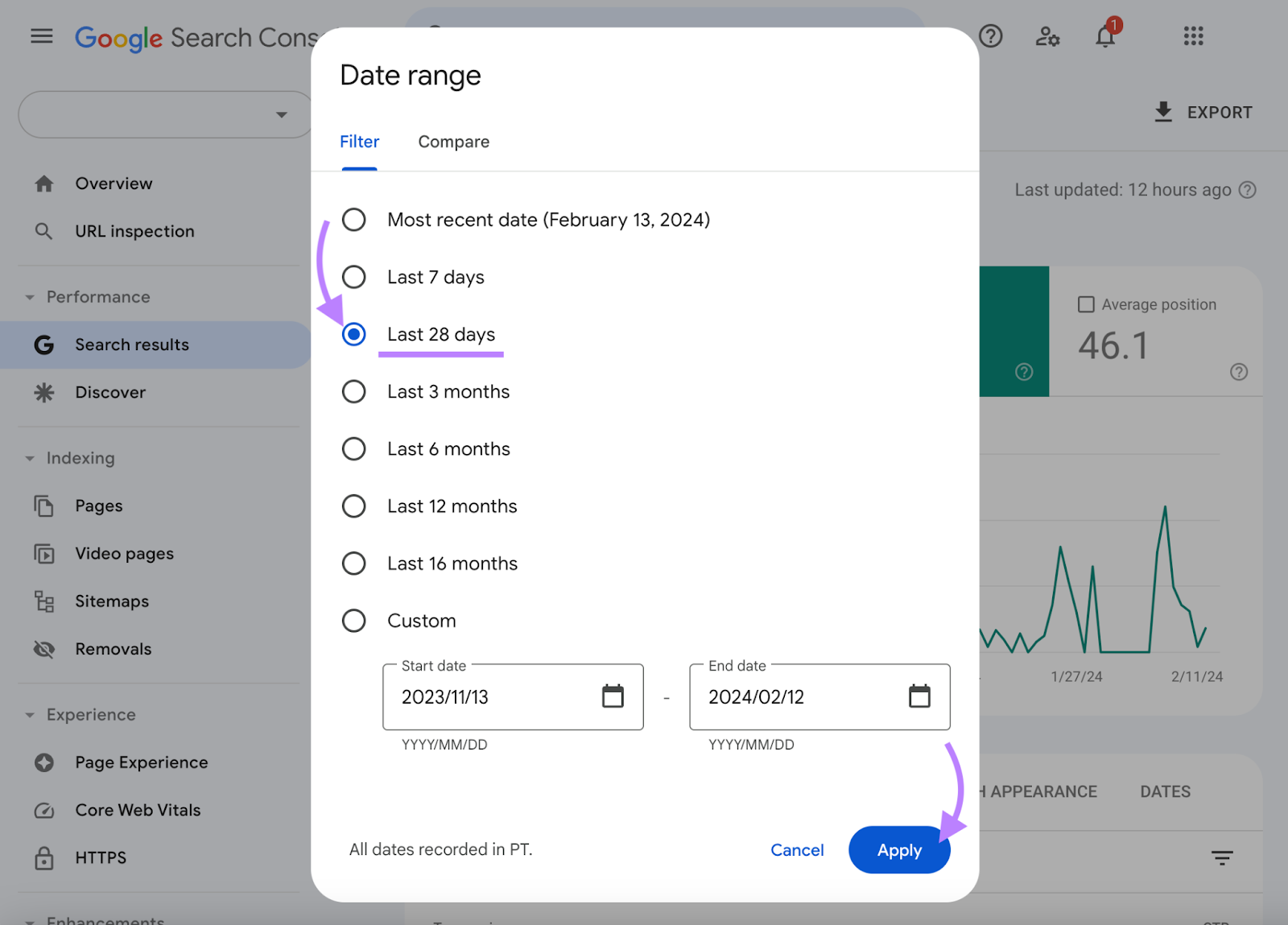The image, oriented in landscape mode, depicts a Google Search Console interface with a form in the foreground. The background showcases a typical Google search results layout.

In the upper left corner of the form, there is a label that reads "Date Range." Directly below, two tabs are visible: "Filter" and "Compare." The "Filter" tab is selected, highlighted in light blue, and underlined.

The form contains eight rows, with the third row notably emphasized. The creator of the image has drawn a purple, curving arrow pointing to this third row, which is also underlined in purple. This row shows the selected filter option, indicated by a blue bullet point, labeled "Last 28 Days." The other filter options listed include:
- Most Recent Date: February 13, 2024
- Last 7 Days
- Last 3 Months
- Last 6 Months
- Last 12 Months
- Last 16 Months

Beneath these options is a custom date range field, which allows users to specify a "Start Date" and an "End Date," shown here as "2023-11-13" and "2024-02-12" respectively, with all dates recorded in PT (Pacific Time).

On the right side of the form, there are two buttons. The "Cancel" button is blue, while the "Apply" button is also blue but features white font. A second purple, curving arrow points towards the "Apply" button, indicating it should be clicked.

The backdrop of the entire scene is the Google Search Console, with the "Search Results" section highlighted.